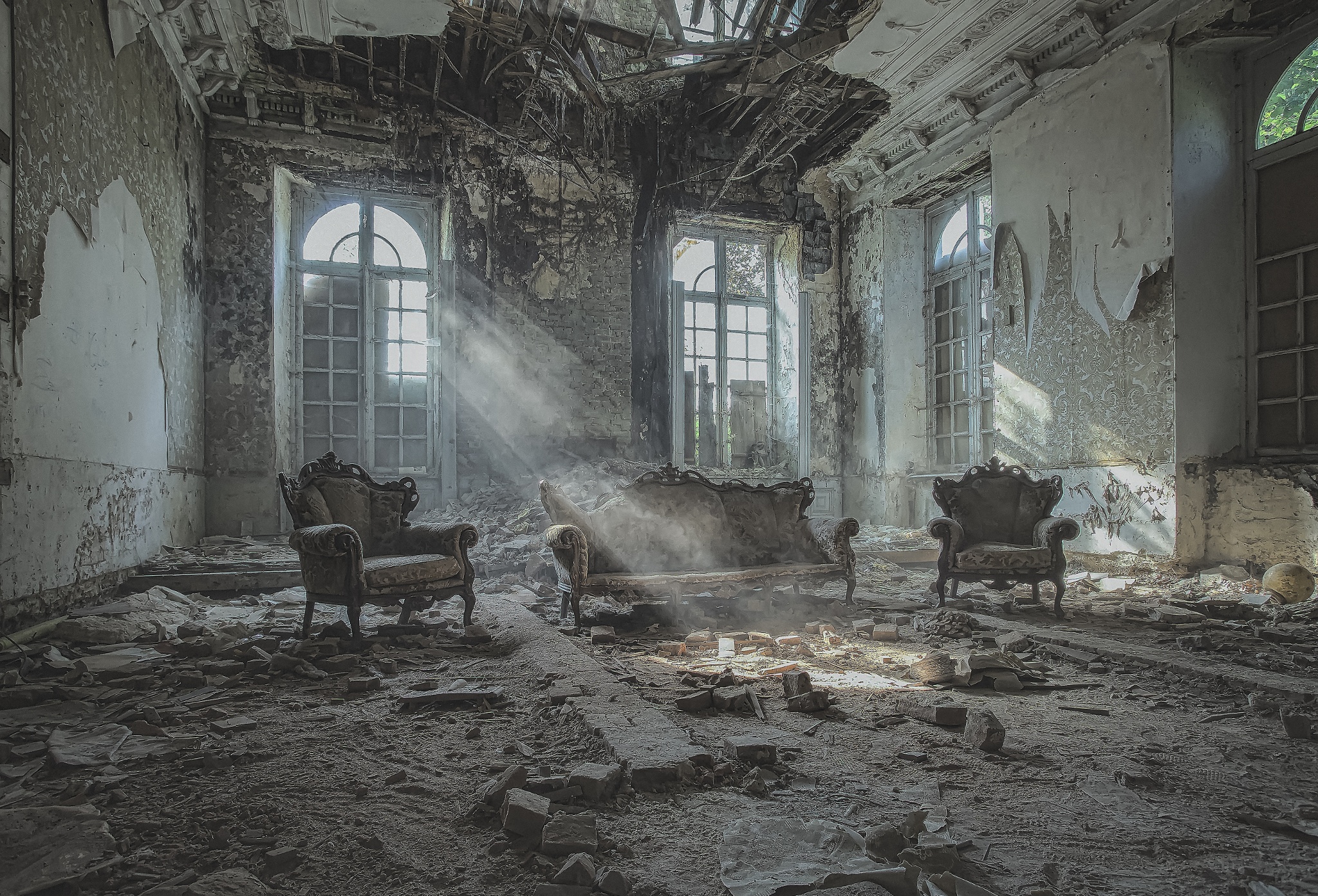This photograph captures the haunting decay of a once grand, now abandoned house. The large room, with a ceiling at least 15 feet high, reveals extensive damage and desolation. The roof is caved in, and broken, boarded-over windows with some missing boards allow rays of light to pierce the gloom, lighting up the dust in the air. The floor is a chaotic landscape of debris, including torn bricks, dirt, and remnants of what might have been an ornate brickwork. The walls are in ruin, with plaster and paint missing, and tattered wallpaper hanging in strips. Despite the devastation, a sense of former opulence persists with the presence of elaborate, ornately designed furniture - a couch and two chairs that appear almost out of place among the wreckage yet retain their decorative charm. Everything, from the furniture to the piles of rubble, is cloaked in layers of dirt and grime, contributing to the eerie atmosphere of this forsaken interior.